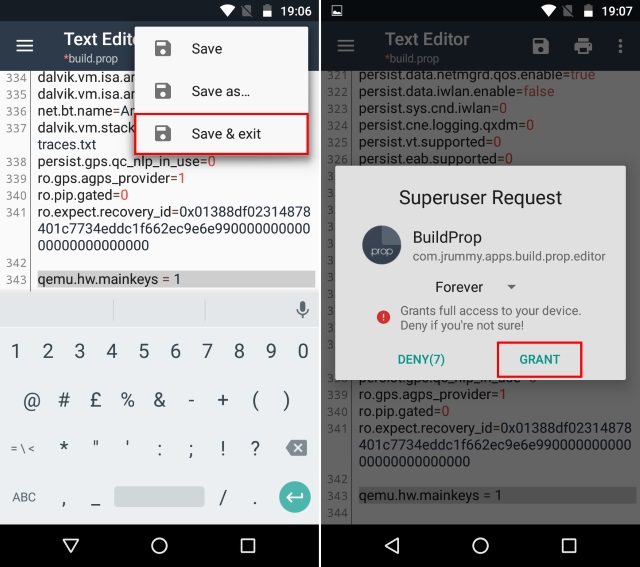A detailed screenshot capture from a tutorial illustrates the step-by-step setup process for configuring a specific page. On the left side, a small pop-up window is prominently displayed, featuring options titled "Save," "Save as," and "Save and Exit" in sequence. Below this pop-up, numerous lines of code are visible, suggesting that coding instructions form part of the tutorial. The keyboard is partially visible at the bottom of the screen, hinting at active user interaction. On the right side, another pop-up window labeled "Super User Request" appears. This window displays instructions pertaining to "build.prop" with a dropdown menu set to "Forever," indicating persistent settings. The message advises users that granting full access will provide complete control over the device while cautioning to deny access if uncertain. A conspicuous "Grant" button is placed to the right, facilitating the user's permission to proceed.